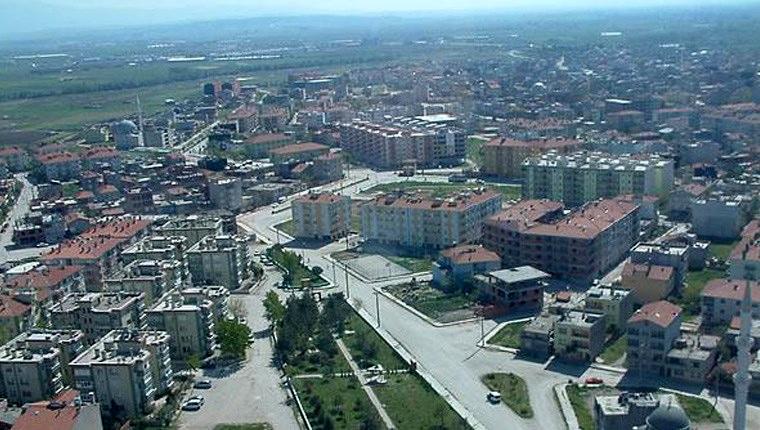The image depicts an overhead view of a sprawling residential area, showcasing an assortment of residential buildings that range from four to perhaps less than ten stories tall, many designed in a typical early 2000s architecture style. The buildings predominantly feature white or brown exteriors, with several having reddish-brown or white roofs. Those with white roofs often appear to have accessible rooftop spaces adorned with plants and shrubbery. Dividing the residential blocks are gray streets, noticeably sparse in traffic, and a van can be seen driving in the foreground. Interspersed between the buildings and streets are green areas filled with trees and grass, adding a touch of nature to the otherwise urban landscape. In the far background of the image, the cityscape fades into a grassland, giving way to a vast expanse of green that stretches towards the horizon, where it meets the sky.